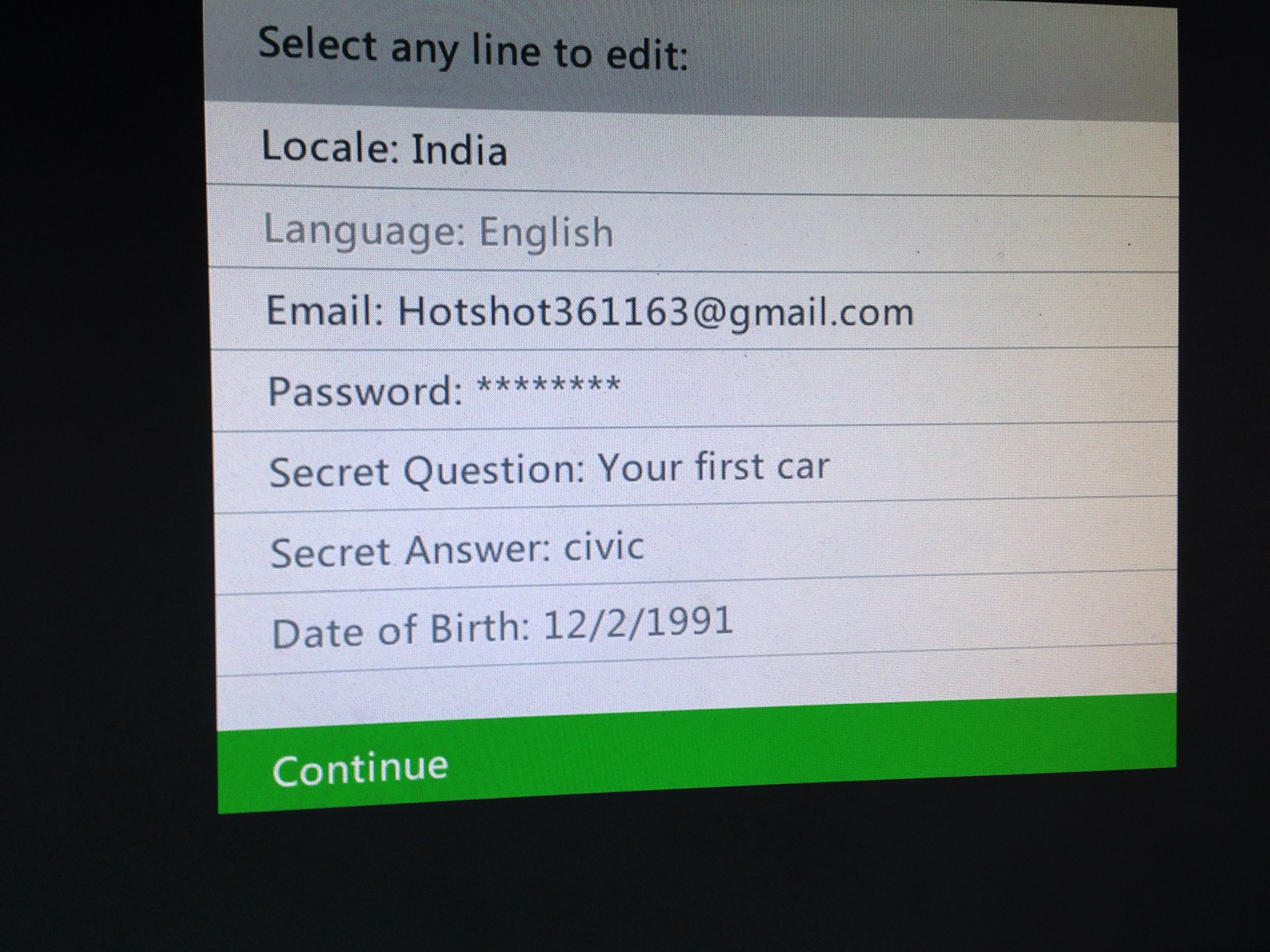The image is a close-up screenshot of a laptop screen displaying a drop-down menu from an application. At the top of the menu, a dark gray rectangular bar features the text "Select any line to edit:". Below this, a white section systematically lists personal details. The locale is "India," and the language is "English." The email is "hotshot361163@gmail.com," and the password is represented by a series of asterisks. The secret question is "Your first car," with the answer "Civic." The date of birth listed is "12-2-1991." At the very bottom, a green rectangle contains the word "Continue." The screen appears to be tilted slightly at an angle, set against an overall dark background.